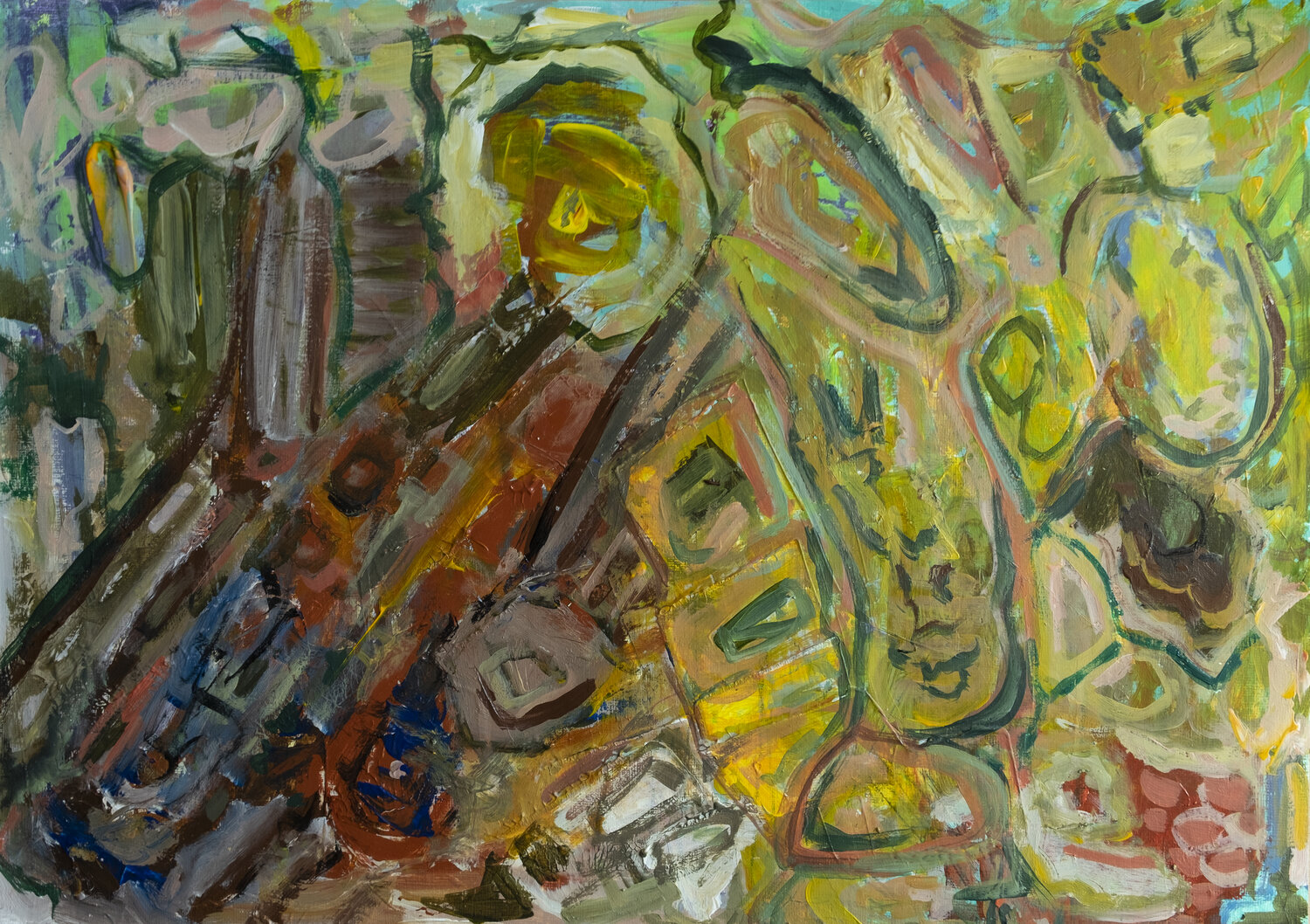This detailed abstract painting is a striking display of conceptual artistry, filling the entire canvas with a rich, heavily textured matte surface, possibly crafted with acrylic paints. The artwork features an array of muted yet vibrant colors that dynamically shift from dark rust reds, deep browns, and navy blues on the left to lighter pastel shades of yellows, light greens, sky blues, and hints of pinks and reds on the right, creating a dramatic contrast. The composition is a blend of geometric shapes such as rectangles and roughly drawn squares, intertwined with organic swirls, ovals, and kidney-shaped forms that evoke a sense of chaos and playful spontaneity. While the image doesn't depict any discernible subject matter, the arrangement of shapes and lines suggests an impressionistic or surreal representation that feels both energetic and vehemently alive. The peculiar orientation, with shapes angled towards the top right corner and extending to the lower left, imbues the painting with a dynamic tension, making it an intriguing visual experience.